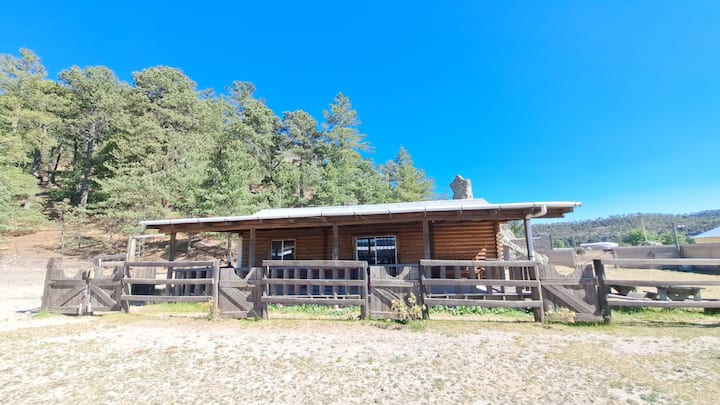The image captures a rustic, one-story log cabin or ranch-style house with a sloping grey roof. The house, constructed of brown wooden logs, features four glass-paneled windows—two prominently visible, and two more subtly placed. Surrounding the house is a sturdy, grey wooden fence that encloses the property. In the foreground, a patch of arid, greyish-beige land, speckled with sparse green grass, stretches before the house. To the left of the scene, tall and sturdy green trees add a natural touch, while to the right, an expansive mountainous region forms a stunning backdrop. The scene, bathed in broad daylight under a bright blue sky, suggests a peaceful rural or farm setting, possibly with an animal enclosure on the right side of the house.